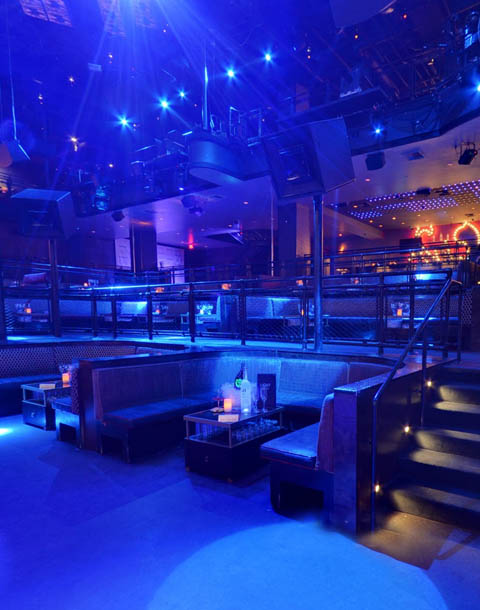The photo captures the interior of a dark, vibrant nightclub filled with an array of bright, neon lights that predominantly cast blue and purple hues across the scene. In the foreground, there's a dance floor leading to a middle ground with curved U-shaped booths equipped with small tables adorned with drinks, candles, and possibly menus. To the right, a black staircase ascends to a bar area complete with additional tables and bar stools. Overhead, numerous spotlights and speakers hang from the ceiling, contributing to the atmospheric club lighting. In the background, the bar area is flanked by various doors, with a stage illuminated by bright orange and yellow neon lights. The entire space is devoid of people, presenting an inviting yet mysterious ambiance.